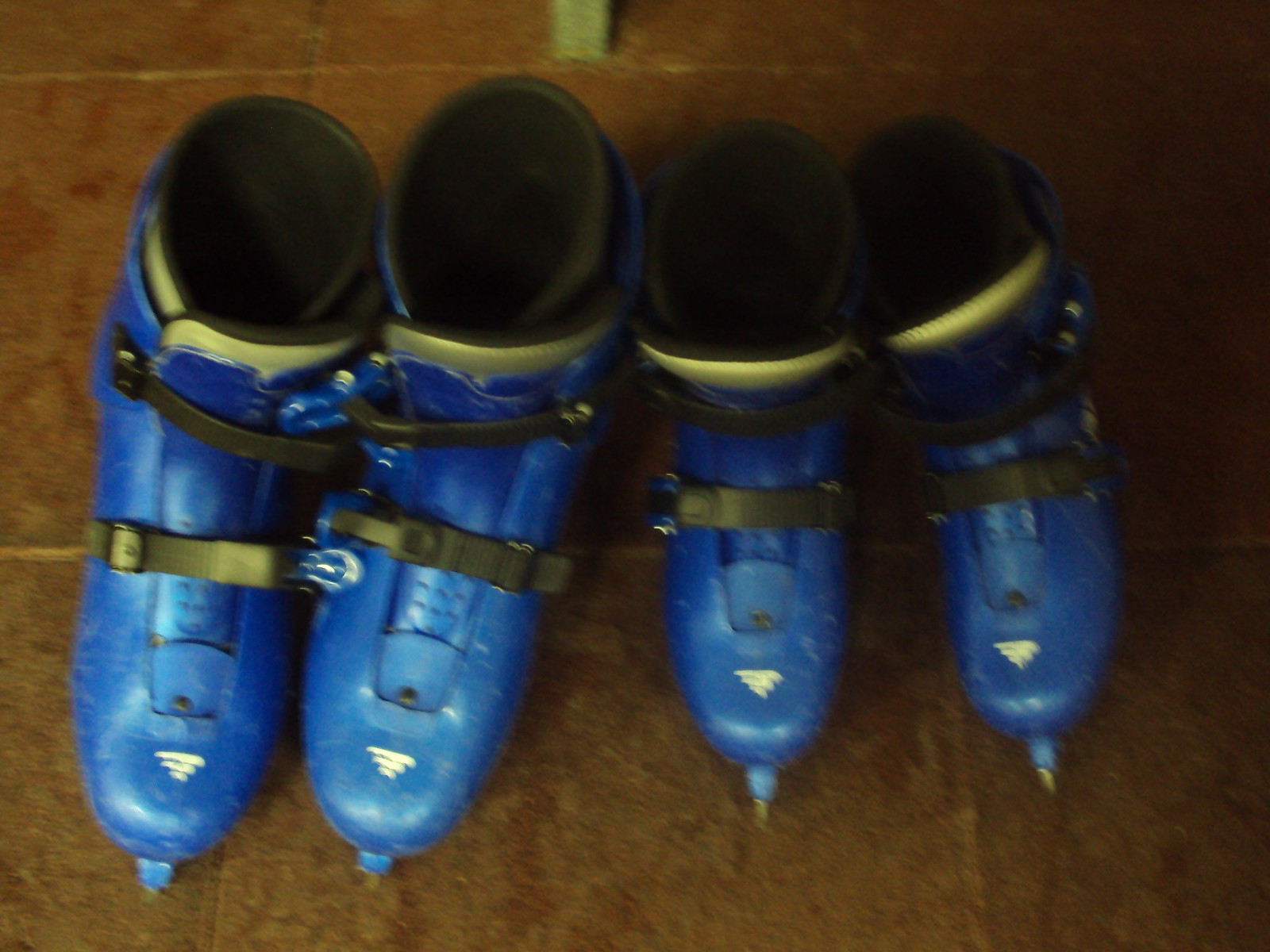The image depicts a slightly blurry, possibly older photograph of two pairs of plastic blue ice skates on a dark brown, likely ceramic tiled floor. The pairs are differentiated by size; the larger pair on the left and the smaller pair on the right, suggesting one is for an older child or adult, and the other for a younger child. Both pairs share identical design features, including black clasps, a silver and black tongue, and a black cushioned interior. The skates exhibit a distinctive golden coloring around the areas where the foot would be inserted, and a triangular design with three white lines on the front. Intriguingly, there's a piece of wooden furniture, possibly a table leg, visible in the background, though it's not clearly identifiable.